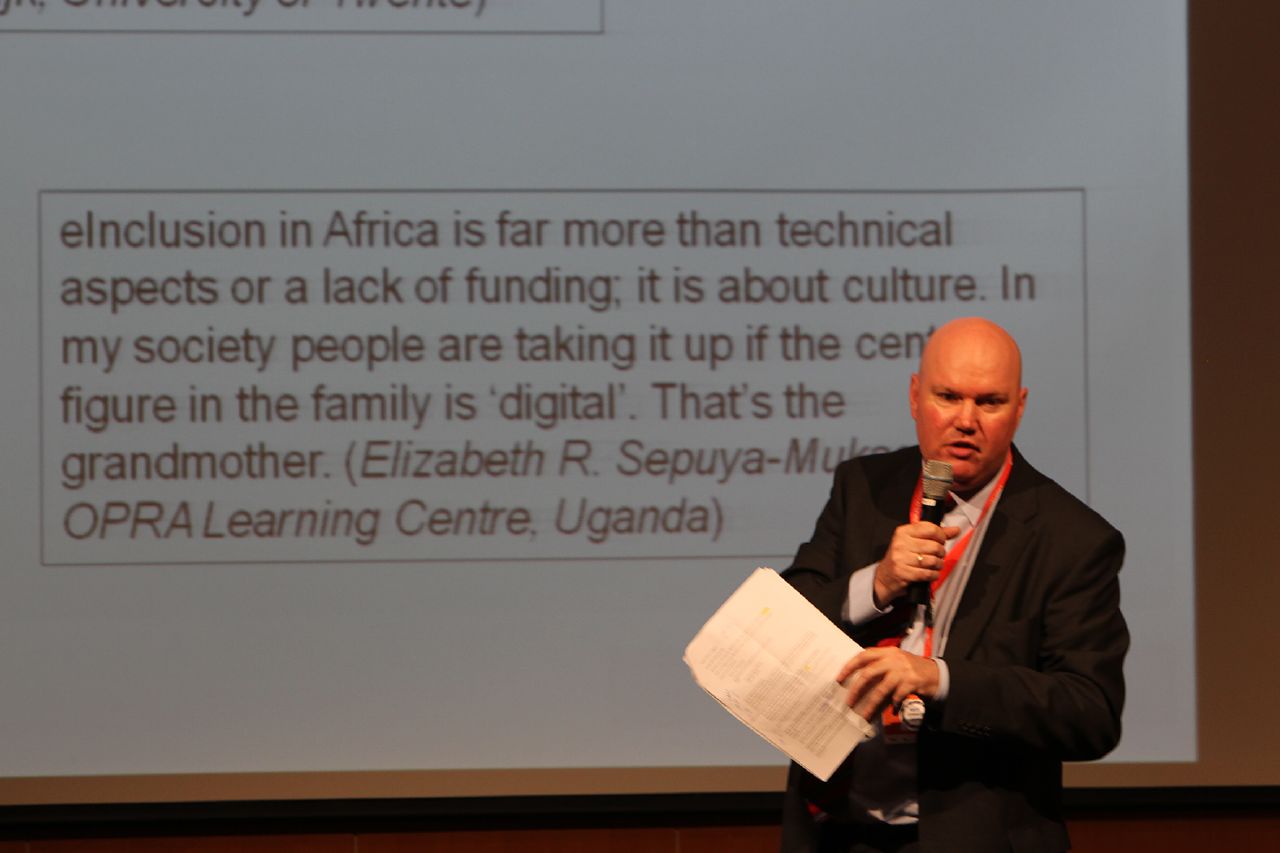A detailed horizontal rectangular image captures a bald, clean-shaven man giving a talk about Africa. He is positioned in the lower right corner, dressed in a white button-up shirt underneath a black suit jacket, with an orange lanyard around his neck. He holds a black microphone in his right hand and several sheets of paper in his left. The backdrop features a large white projector screen surrounded by a brown border. Displayed on the screen is a slide with a text box outlined in black. The text reads: "e-inclusion in Africa is far more than technical aspects or a lack of funding. It is about culture. In my society, people are taking it up if the center figure in the family is digital. That's the grandmother." The slide includes the credit "Elizabeth R. Sepua Dash, OPRA Learning Center, Uganda," though the man's body partially obscures some of the text.